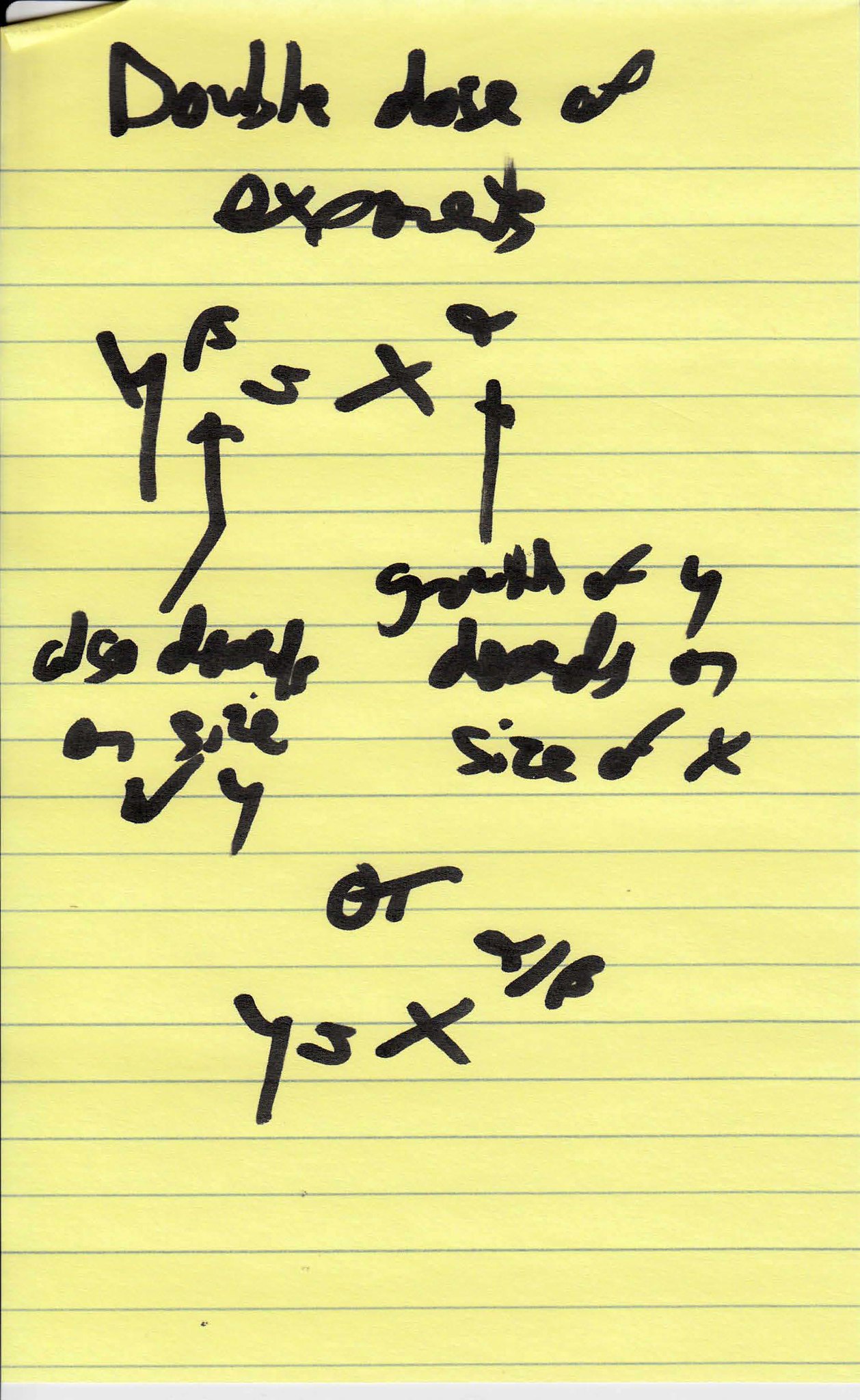A detailed photograph showcases a yellow sheet of paper from a legal pad, characterized by light blue horizontal lines running evenly across its surface. At the very top, the upper-left corner is slightly folded down. The writing on the paper is done in thick black marker, giving it a bold appearance. The text begins at the top, with the ambiguous phrase “double dose of exponents” or something similar suggesting a possible mathematical context. Below this, the sheet appears to contain a math problem, featuring symbols such as a "7," a "B," a "3," and a multiplication symbol. An anomalous drawing resembling a small fish points to the left. Several arrows indicate upward to a section that provides additional instructions or descriptions, though the exact wording is difficult to decipher. One part of the text reads “size equals Y,” while another mentions “size of X or equals X.” Near the bottom center of the page, the letters “OT” stand out, followed by another sequence of symbols that includes a "7," a "3," an "X,” a fish-like doodle, a slash, and a "B." The overall scene suggests the page contains someone's handwritten notes, possibly from a math class, with various doodles and annotations that add to its complexity.